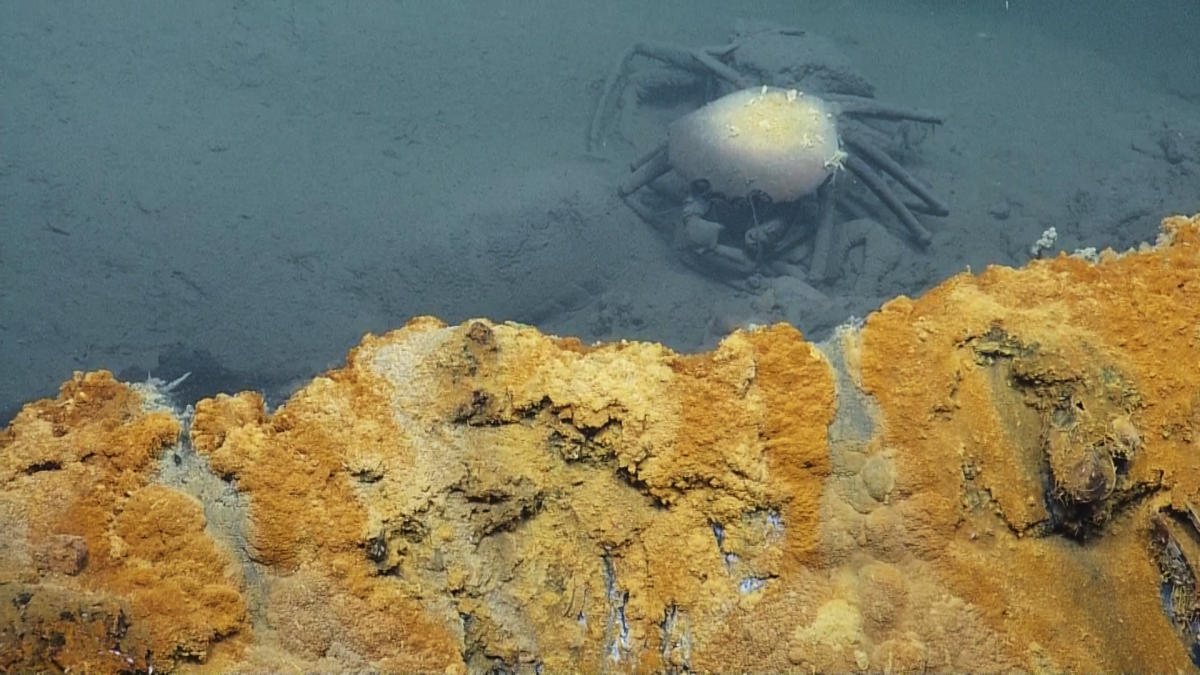An aerial photograph captures a beach scene where the shoreline meets a body of water. The bottom portion of the image showcases a mix of brown sediment and clay-like rocks, also containing patches of orange hues, stretching across the shore. The sediment varies in size from smaller clumps on the left to larger ones on the right. As the terrain transitions into the water, the top half of the photograph reveals a dark blue, somewhat murky water body, complete with visible sandy or clayish materials beneath due to its clarity, suggesting fresh water. Notably, there's a peculiar white sea creature in the water resembling a crab, distinguished by its eight legs and two black eyes. It appears to be moving over some scattered sticks present in the water. This white creature's unique coloration and presence amidst the natural elements of the beach and water create an intriguing focal point in the otherwise typical coastal scene.